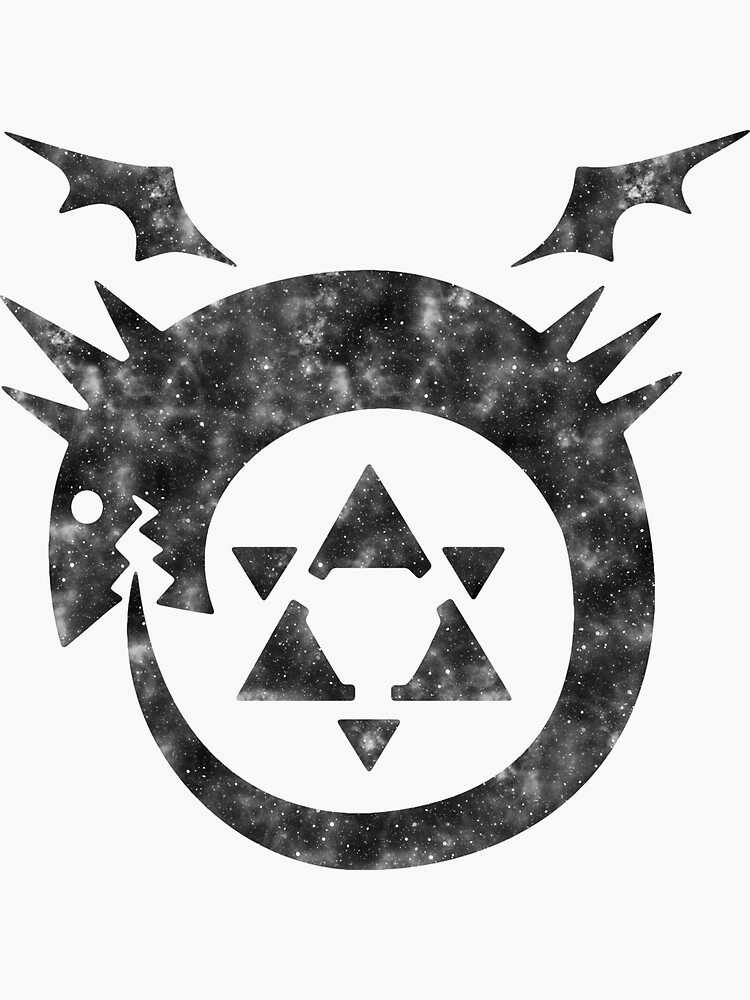A minimalist black and white design dominates this image, with a predominantly white background that makes up most of the composition. The stark contrast is provided by an intricate and detailed black-and-gray logo at the center, which becomes the focal point of the artwork. The logo features a stylized dragon, almost forming a circle as if it is on the verge of consuming its own tail. This dragon is depicted with pronounced spikes and prominent black wings, adding a dramatic flair to the image. Inside the dragon's circular form lies a complex geometric pattern: two interlocked triangles that are further divided into smaller triangular fragments, creating an intricate and visually engaging centerpiece within the larger circular logo.